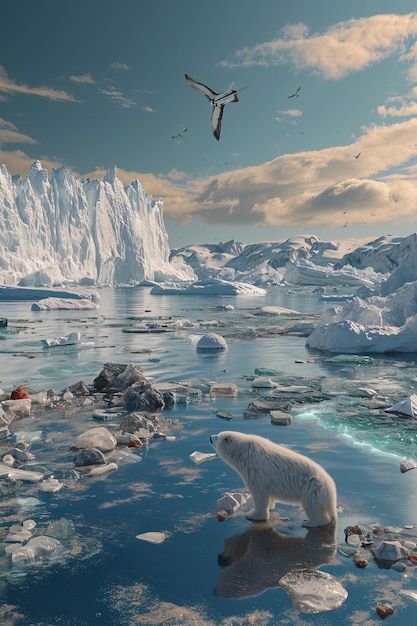This illustration depicts a serene yet evocative Arctic scene. In the foreground, a lone polar bear stands on a seemingly ice-covered body of water, where reflective layers reveal scattered stones peeking through the ice. The bear gazes into the distance under a sunny sky adorned with light blue hues and white, shadowed clouds. Sea birds circle above, adding life to the otherwise stark landscape. Large glaciers and floating chunks of ice, complete with the bear's reflection, are strikingly evident. Amidst this intricate glacial terrain, patches of detritus and beige-colored trash punctuate the icy expanse, hinting at underlying environmental concerns. The surrounding scene is framed by snow and rocky formations, emphasizing the contrast between the natural beauty and subtle intrusion of human impact.